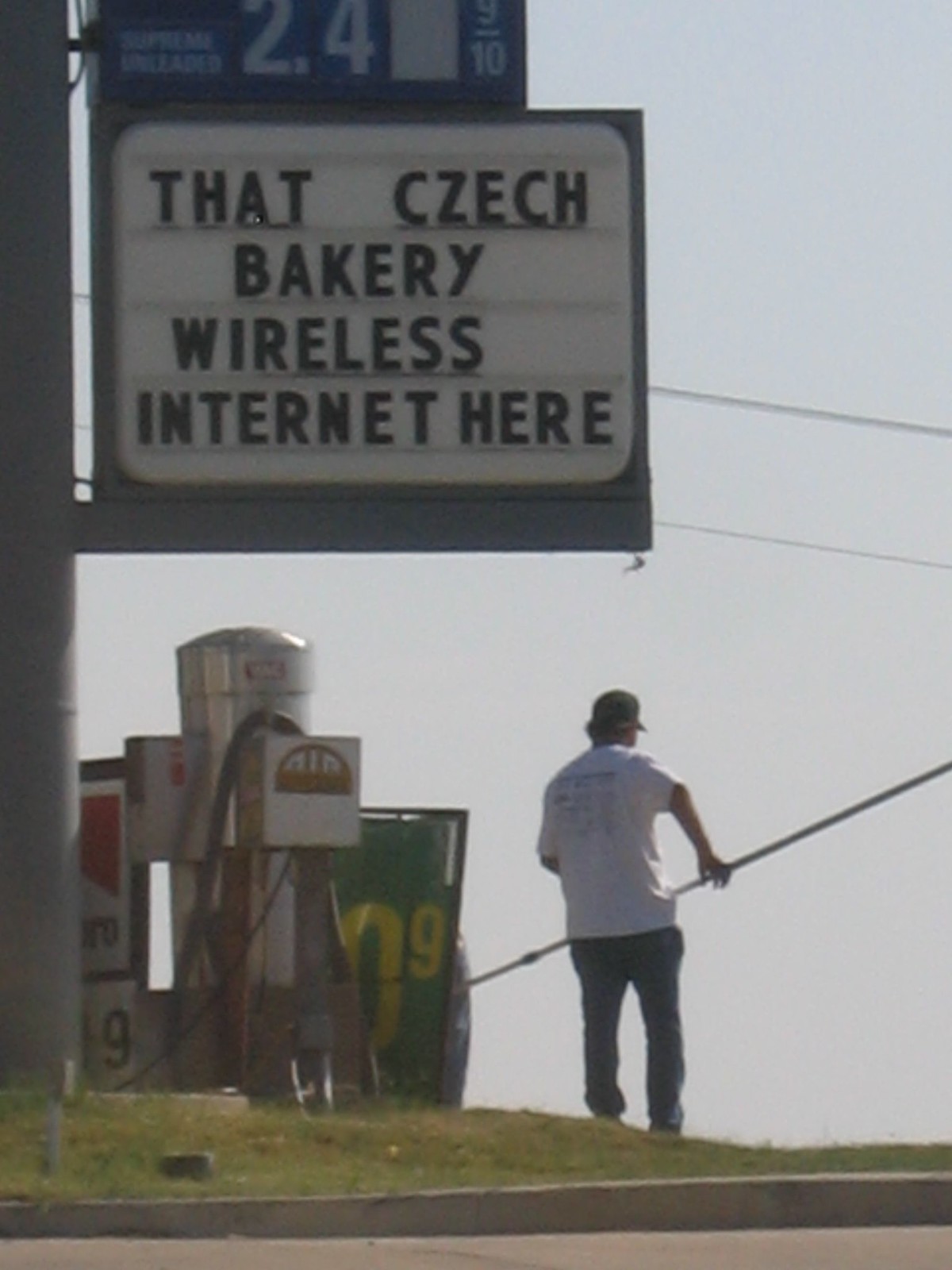In this photograph, a man is seen from behind, standing beneath a marquee sign at what appears to be a gas station. He is dressed in jeans, a white shirt, and a baseball cap, and he holds a long pole, likely used for changing the letters on the marquee. The marquee reads "Czech Bakery Wireless Internet Here." Above the marquee is a gas station sign displaying fuel prices, with "Super Unleaded $2.40" clearly visible. Next to the man, a gas pump stands, further indicating the gas station setting. The scene captures a candid moment of the man amidst his likely task of updating the marquee, his back turned to the photographer, emphasizing the routine nature of his work.